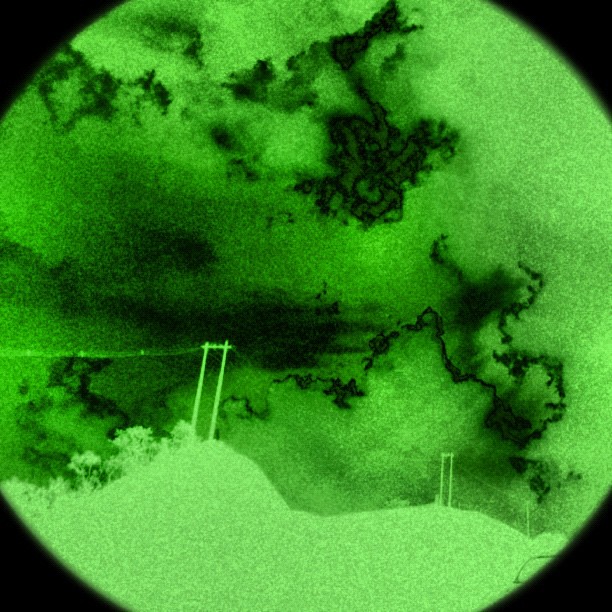The image is a color photograph with special effects, presenting a circular view through a green lens, set against a black background. The circular frame, which gives the photo a distinctive look, is green with a mix of neon tones and black grainy streaks creating a swirling, stormy effect in the sky. The circular image appears to be slightly cropped at the edges within a square format. Dominating the top and middle sections of the circle are dark, swirling clouds, adding to the stormy atmosphere. Beneath the clouds, the ground features a profile of a hillside or heaps of sand, dotted with small green plants or weeds. Prominently, three tall electricity poles stretch across the scene, their silhouette lined with wires connecting them. Overall, the image combines natural elements with industrial ones, all viewed through a vivid, colorized lens effect.